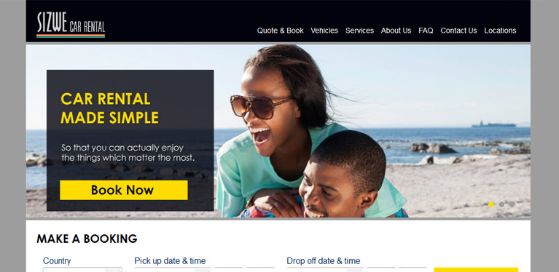The image portrays a detailed webpage layout for a car rental service. At the top, there is a black bar, within which the brand name "Sizwe Car Rental" is prominently displayed in white text in the left corner. Directly beneath the name, a series of horizontal stripes in red, yellow, and green hint at a possible connection to Jamaican colors, inferring a vibrant and welcoming identity.

To the right of the brand name, the navigation bar features several menu options: "Quote & Book," "Vehicles," "Services," "About Us," "FAQ," "Contact Us," and "Locations," providing easy access to various informational and functional sections of the site.

The central portion of the page is dominated by an engaging image of a smiling couple, comprising a man and a woman, both of African descent, enjoying a picturesque day at the beach, exuding a sense of joy and relaxation. The woman is notably wearing glasses, and their expressions and the sunny setting suggest they are on a delightful vacation.

Adjacent to the couple's image is a prominently placed text box that reads, "Car rental made simple, so that you can actually enjoy the things which matter the most." Below this reassuring message, a vibrant yellow "Book Now" button in black lettering invites users to proceed with their rental booking.

Beneath the central image, there is a functional "Make a Booking" section, enabling users to input crucial details such as their country, pickup date and time, and drop-off date and time. An accompanying yellow button likely serves to initiate the search for available vehicles.

Despite the right portion of the page being partially cut off, the visible elements effectively communicate the website's purpose and user-friendly design, underscored by the happy couple enjoying their vacation backdrop under sunny skies.